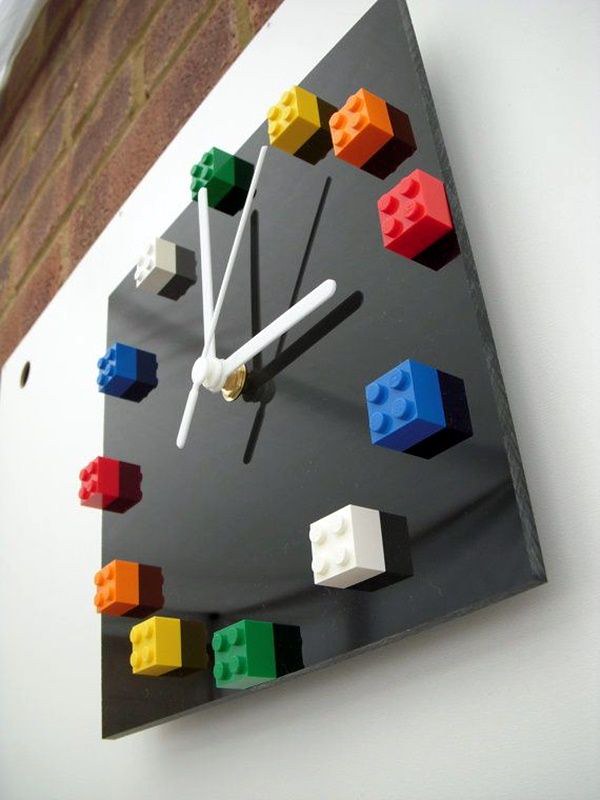This image features a striking wall clock that is prominently displayed on a white wall. The clock is square-shaped, with a sleek black clock face that contrasts sharply against the bright white surroundings. The clock’s hands are white and are attached to the center via a golden metallic hub, which stands out against the black background.

Intriguingly, the clock face is embellished with 2x2 Lego blocks in various vibrant colors, which replace the traditional numbers. At the topmost position is a green square, followed by a yellow square, then an orange one as we move in a clockwise direction. This sequence continues with red, blue, white, green, yellow, orange, red, blue, and white Lego squares forming the entirety of the clock’s hour markers.

The clock hands are in dynamic positions, indicating time amidst a colorful assembly of Lego blocks. The shortest, thickest hand (denoting hours) points to the rightmost red square. The slightly longer, thicker hand (denoting minutes) targets the uppermost green square. Meanwhile, the thinnest and longest hand (denoting seconds) points towards the adjacent right yellow square. Notably, the clock hands cast delicate reflections on the clock face, adding depth to the image.

Additionally, the environment surrounding the clock adds character to the scene. Above the white wall is a contrasting reddish brick wall. To the left of the clock, a small hole is visible within the white wall. The space appears to be well illuminated, enhancing the vividness of the colors and the details of the surroundings.